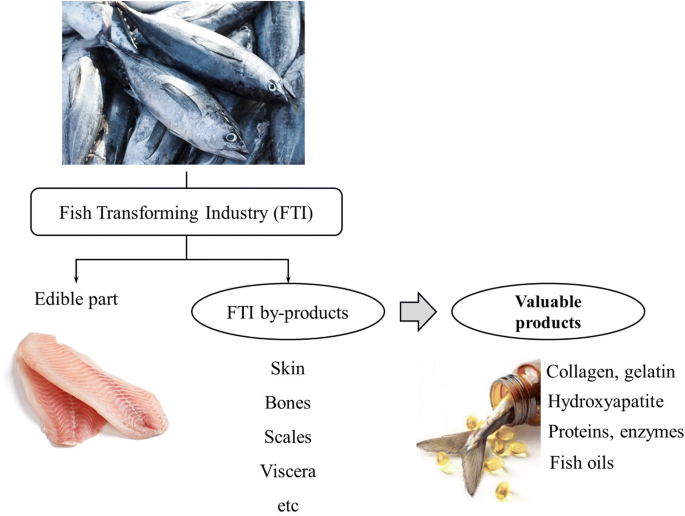This image is a detailed, color-illustrated flowchart titled "Fish Transforming Industry (FTI)." It illustrates the transformation of fish into various products. Starting in the upper left, there's a black and white photograph of several medium-sized, silver-colored fish stacked in a pile. Underneath this image is a horizontal text box labeled "Fish Transforming Industry (FTI)." An arrow from this text box points downward and splits into two branches: one to the left and one to the right.

The left branch is labeled "Edible Part" and features a photo of two pink fish fillets, one stacked on top of the other. The right branch is labeled "FTI By-products" and lists components such as skin, bones, scales, and viscera. Following this, a thick gray arrow points to another section labeled "Valuable Products." Here, there's an image of a fishtail protruding from a jar lying on its side, with clear-colored pills scattered underneath. Adjacent to this image is a list of items derived from the fish by-products, including collagen, gelatin, hydroxyapatite proteins, enzymes, and fish oils.

The flowchart is designed with a clean white background typical of web page graphics, and utilizes colors like tan, gray, yellow, black, and pink to distinguish various elements. This diagram serves as an informative visual guide to the fish transformation process, from initial raw fish to final valuable products used in homes.